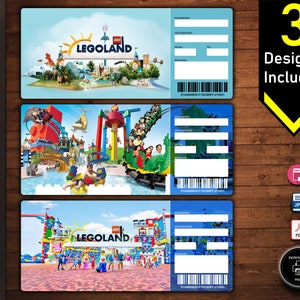The image features a brown wooden table with horizontal planks that have a dark textured grain. Placed on the right side of the table are three rectangular cards, each laid out horizontally.

The top card has a light blue background with dark blue text that reads "LEGOLAND." Above the text on the left side is an illustration of a half sun. The background of the card is adorned with images of dinosaurs. There is a designated area on the right side of the card for entering a name, phone number, and other relevant details.

The middle card showcases a playful scene with LEGO characters. It depicts a castle or playground setting, featuring a green and yellow dinosaur-themed roller coaster with children and adults riding it.

The bottom card also has "LEGOLAND" written on it. It illustrates people walking and playing on brown sand. The sky in this scene is blue with white clouds. Additional icons are slightly visible on the right side of this card. A black ribbon with yellow text at the top right corner reads "Number 3," and below that, white text states "Design Inclusive."